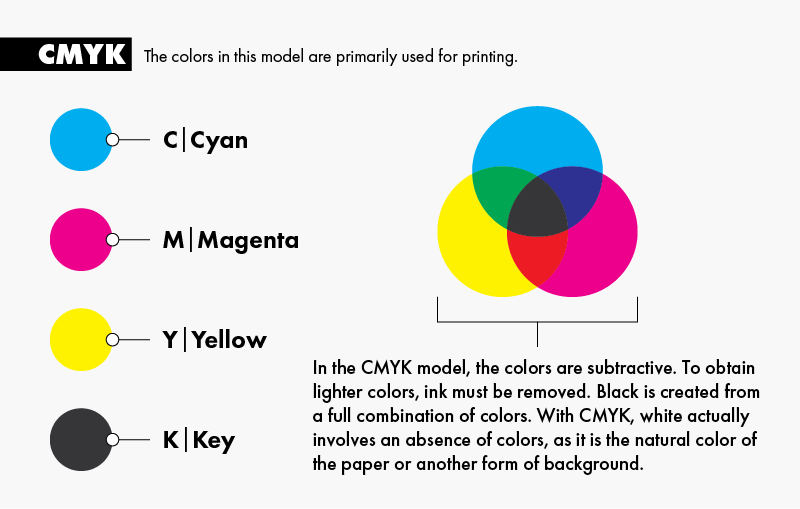This image features a detailed diagram explaining the CMYK color model used primarily for printing. At the top left, the text reads "CMYK," followed by the explanation "The colors in this model are primarily used for printing." Below that, the individual CMYK colors are illustrated with corresponding letters and circles: a blue circle labeled "C" for Cyan, a pink circle labeled "M" for Magenta, a yellow circle labeled "Y" for Yellow, and a black circle labeled "K" for Key. To the right of these circles, there is a diagram showing the overlapping colors: cyan and magenta overlap to produce a dark blue, magenta and yellow create a reddish color, and cyan and yellow form green, with all three overlapping in the middle to illustrate the color black. Underneath, additional text explains, "In the CMYK model, the colors are subtractive. To obtain lighter colors, ink must be removed. Black is created from a full combination of colors. With CMYK, white actually involves an absence of colors as it is the natural color of the paper or another form of the background."